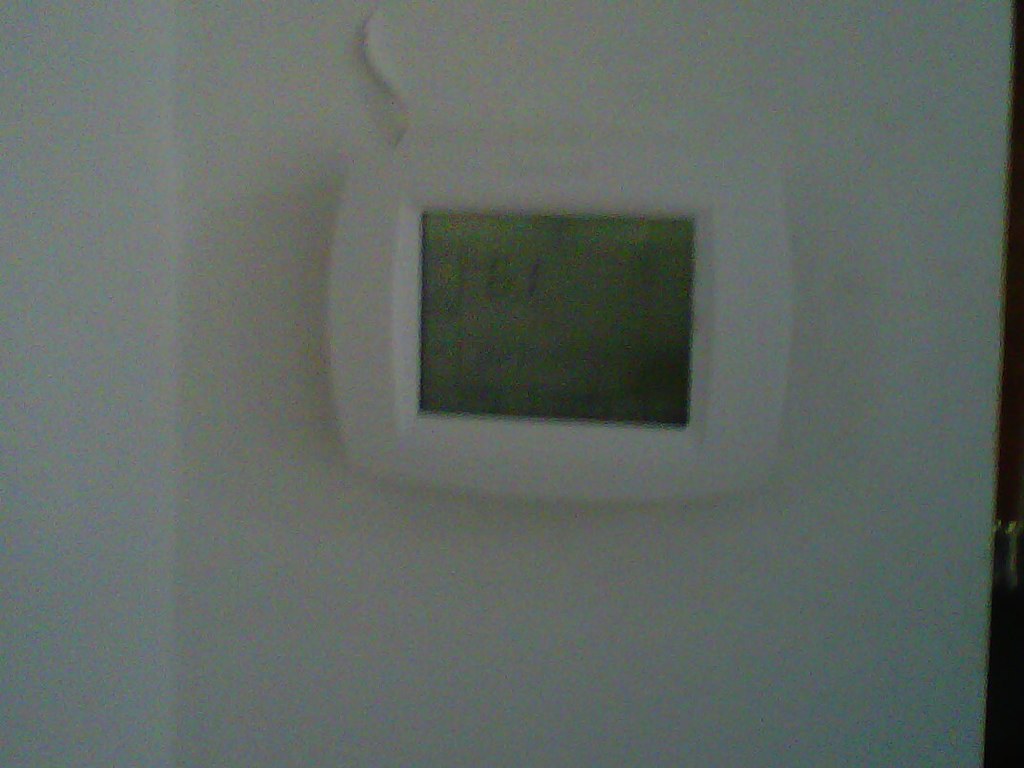Close-up of a white thermostat mounted on an off-white wall, captured in extremely low quality. The pixelated image barely reveals the thermostat's typical features such as an LCD screen at the center. Along the far right edge, beyond the wall, is a dark area indicating it’s not part of the wall. In the lower right corner, a shiny, metallic object is vaguely visible, though indistinguishable due to the poor resolution. The pixelation—likely from using a low-megapixel camera or excessive copying—renders the numbers and writing on the thermostat unreadable.